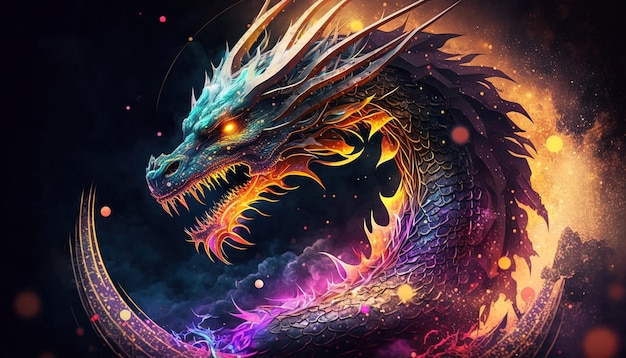The digital painting or 3D rendering depicts a vividly detailed dragon’s head and upper neck, emerging from a rich, textured backdrop. The dragon's neck is adorned with scales in vibrant hues of purple, blue, and orange, transitioning to a predominantly blue head with long, yellow horns extending from the back. Its brilliant, glowing orange eyes and large, jagged teeth add to its fierce appearance. Feathered with spiky ridges, the dragon’s neck appears luminous, as if lighting up the surrounding space. The background contrasts sharply, featuring a stylized orange sky with various circular motifs and white specks, resembling celestial bodies against which dark, stormy clouds gather to the left. The very top left corner of the image fades into complete black, providing a dramatic backdrop. Additionally, the dragon’s partially visible wings tip into the frame's bottom corners, completing this fantastical and vibrant portrayal.